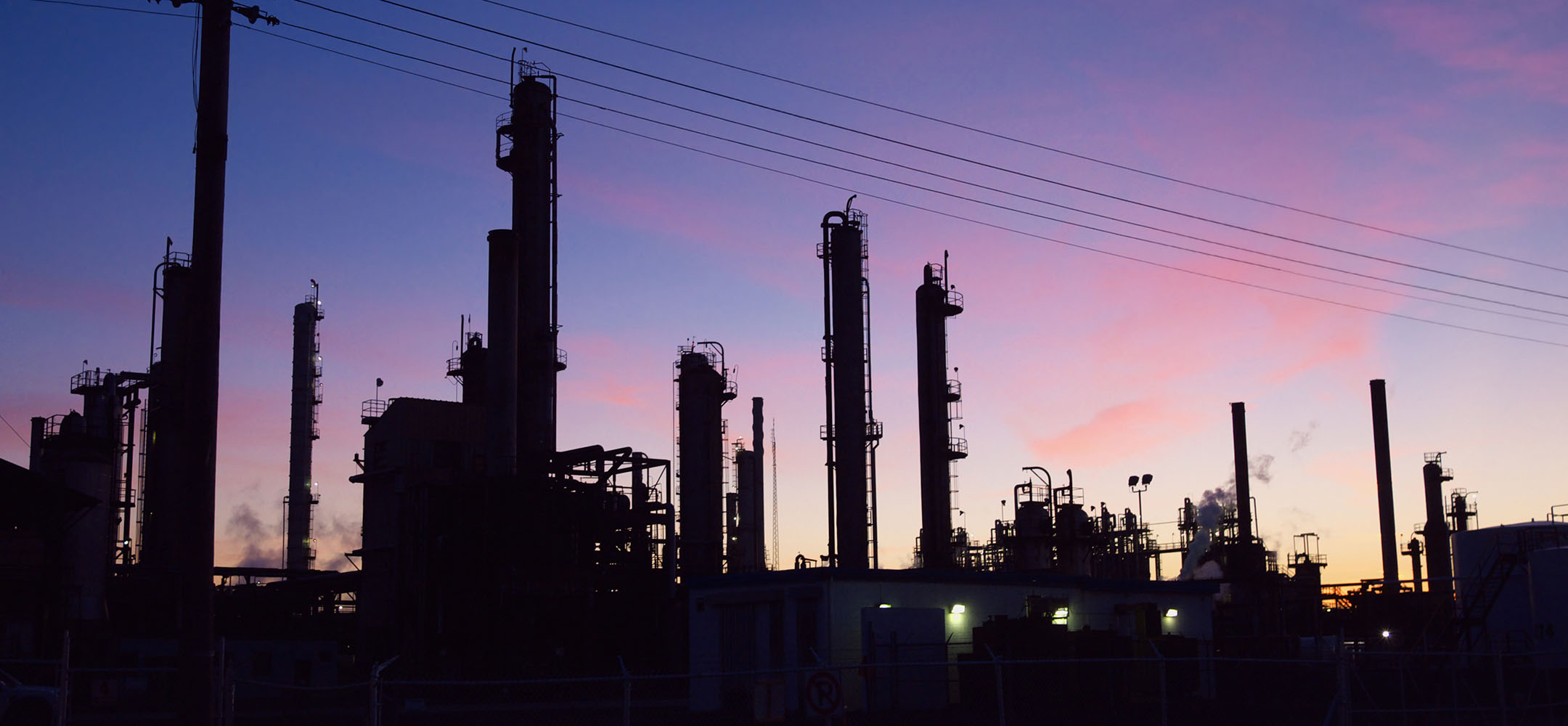This is a night scene photograph of a large industrial plant, likely an oil refinery or chemical plant, captured at sunset. The plant is depicted in a dark silhouette, featuring a complex array of tall towers, stacks, and intricate frames of machinery. The bottom edge of the photograph reveals industrial lighting emanating from the windows of the base structures, highlighting the plant's significant scale. The sky behind the plant is a picturesque gradient of deep blues transitioning into purples, pinks, and peaches, with hints of apricot yellow near the horizon, indicating the sun has not fully set. A set of four power lines stretches diagonally from the upper left to the mid-right of the frame. Wisps of smoke, tinged violet by the setting sun, rise from various stacks, adding to the scene's industrial yet serene ambiance. The absence of people in the image, along with the meticulous silhouette details, emphasizes the vastness and complexity of the refinery against the vivid, dusky backdrop.